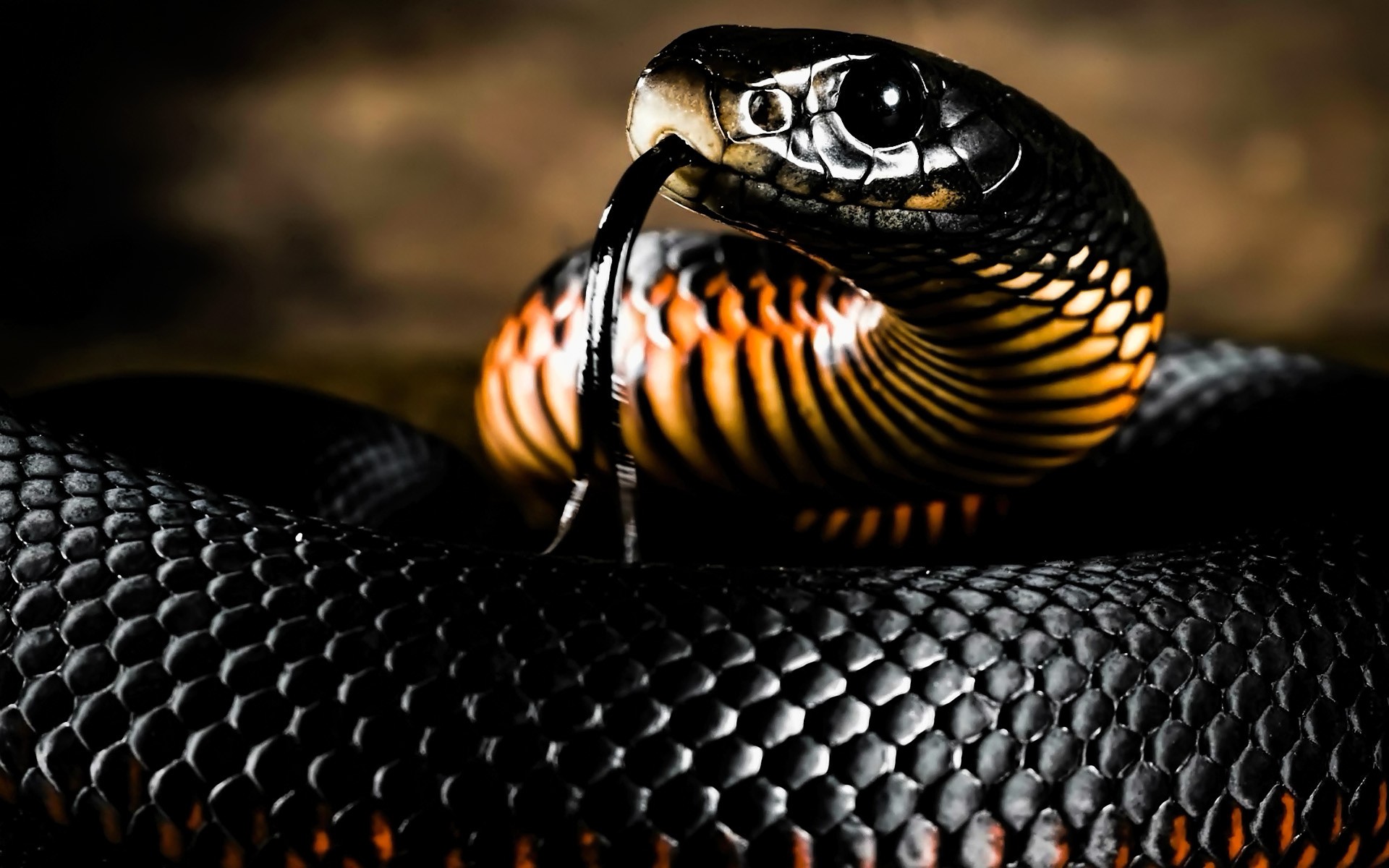In this close-up photograph, a large, predominantly black snake with a striking orange and yellow underbelly is depicted. The snake's shiny black scales glisten, while its orange underside features distinctive black stripes. It is coiled, with its head positioned towards the top center of the image. The snake's long, black forked tongue protrudes from its mouth, and its solitary black eye — adorned with lighter reflections — is prominently visible along with its nostril. The background, a soft brown hue, is blurred to keep focus on the snake. The scene emphasizes the snake's unsettling yet fascinating presence, showcasing its potentially venomous nature.